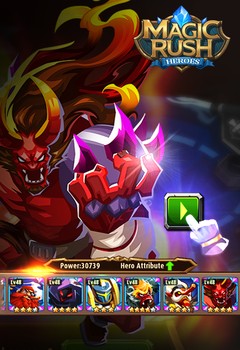The image is a vibrant cartoon graphic with the title "Magic Rush" displayed prominently in the top right corner. Below the title, there is a green play button illustrated with a small white pointing finger, indicating it as an interactive element. Underneath this button, the text reads "Power 3739 Hero Attribute," accompanied by a green arrow.

The central figure in the main frame is a menacing red-horned demon with gleaming gold horns, white snarling teeth, and an intense expression. His hand is clenched over a gray ball, drawing attention to his formidable presence. Surrounding him are a series of character portraits:

1. A red-bearded man with four stars beneath his image, signifying his level or power.
2. A black-cloaked figure with sinister red eyes and mouth, also boasting four stars.
3. A character in a silver and yellow helmet, rated at three stars.
4. A yellow-haired, red-skinned monkey, distinguished by an impressive five stars.
5. A whimsical Pinocchio-like figure, rated at three and a half stars.
6. The red-horned demon, consistent with the main frame figure, also carries a four-star rating.

Each character is depicted with intricate details, emphasizing their unique attributes and power levels, contributing to the dynamic and adventurous theme of the game "Magic Rush."